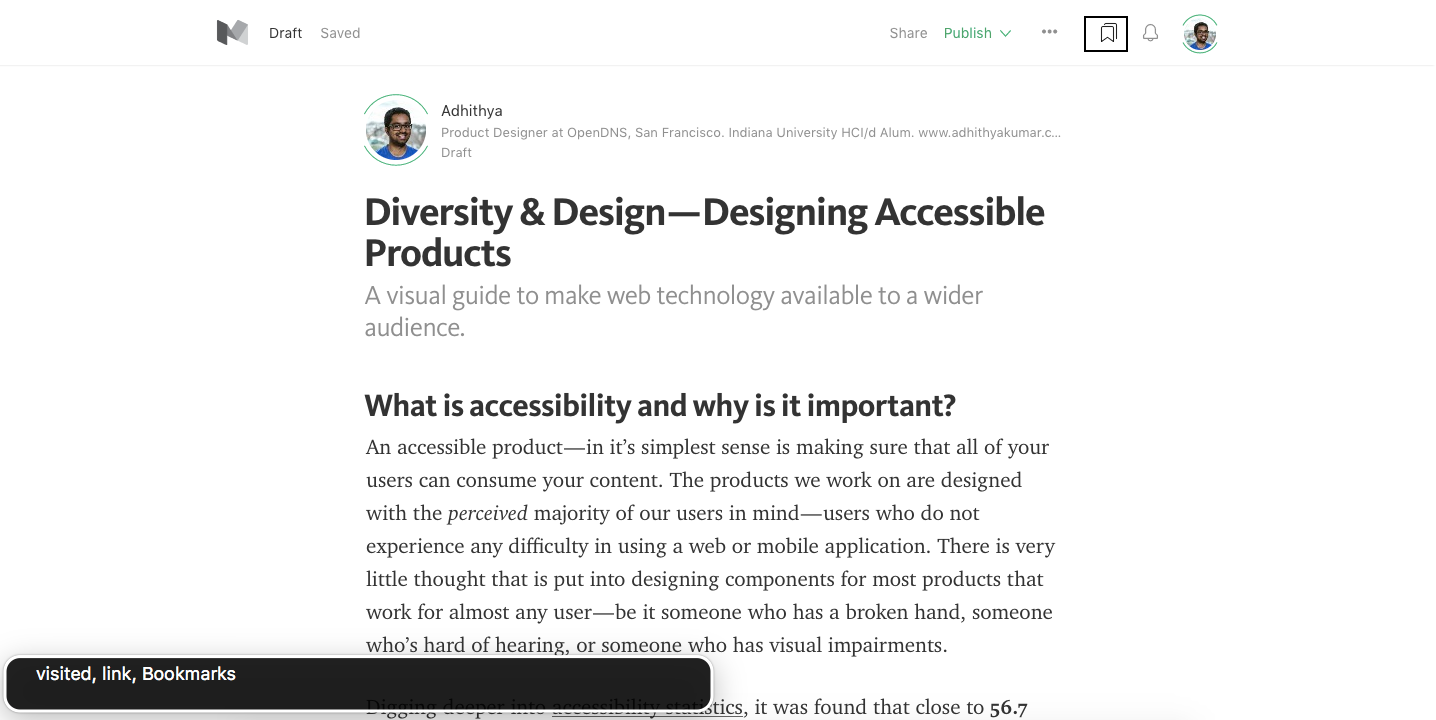This image is a detailed screenshot of a text editing interface on a blogging platform, identifiable by its "M" logo. The platform appears to function as a pay-per-view service, though the specific name isn't recalled. In the user interface, the message "draft saved" is displayed prominently along with options to "share" and "publish," though the "publish" button is notably not highlighted in green, suggesting it's inactive. Other interface elements are rendered in gray or black.

In the upper right corner, there are bookmark icons and a user profile photo, which shows a bespectacled Indian gentleman believed to be Ad Hithaya. His profile details reveal that he is associated with product design and OpenDNS, based in San Francisco, and an alumnus of Indiana University, HC (the specific program or designation is unclear). His profile also includes a link to his personal website.

The article displayed is in draft form, titled "Diversity in Design: Designing Accessible Products," with a subtitle that reads "A visual guide to making web technology available to a wider audience." The introduction poses the question, "What is accessible and why is it important?" and begins with an explanation: "An accessible product, in the simplest sense, ensures that all your users can consume your content. The products we develop are often designed with the perceived majority in mind. Users experience no difficulty using the web or mobile applications, but little thought is given to web design and components that can work for nearly any user, whether they have temporary or permanent disabilities such as a broken hand, hearing impairment, or visual challenges."

Additionally, there is an overlay rectangle in the bottom left corner indicating "visited link and bookmarks." The rest of the article is not visible in the screenshot.